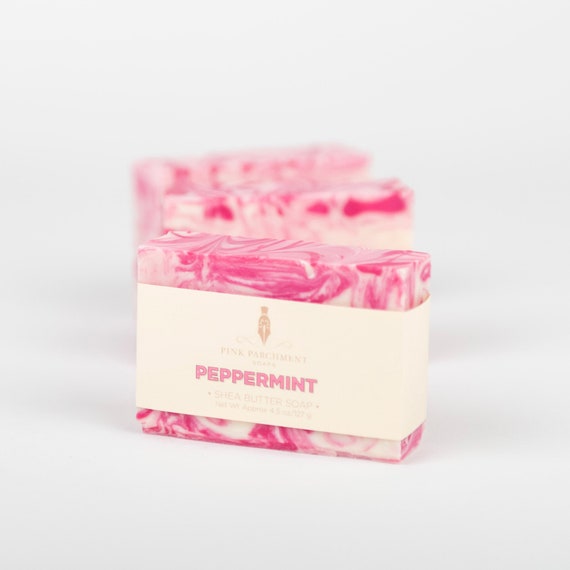The advertisement image features three bars of peppermint shea butter soap displayed on a flat, white surface with subtle shadows against a clean, white or slightly grayish background. The bar of soap closest to the front has a noticeable tilt to the left, while the two bars behind it are progressively more blurred and tilted to the right. Each soap bar is wrapped in a thin, beige or white paper packaging that prominently displays a logo along with the text "pink parchment peppermint shea butter soap." The soap itself is a striking pink and white marbleized pattern, with the front bar showcasing the details about the product's weight and size, though the finer text remains unreadable.